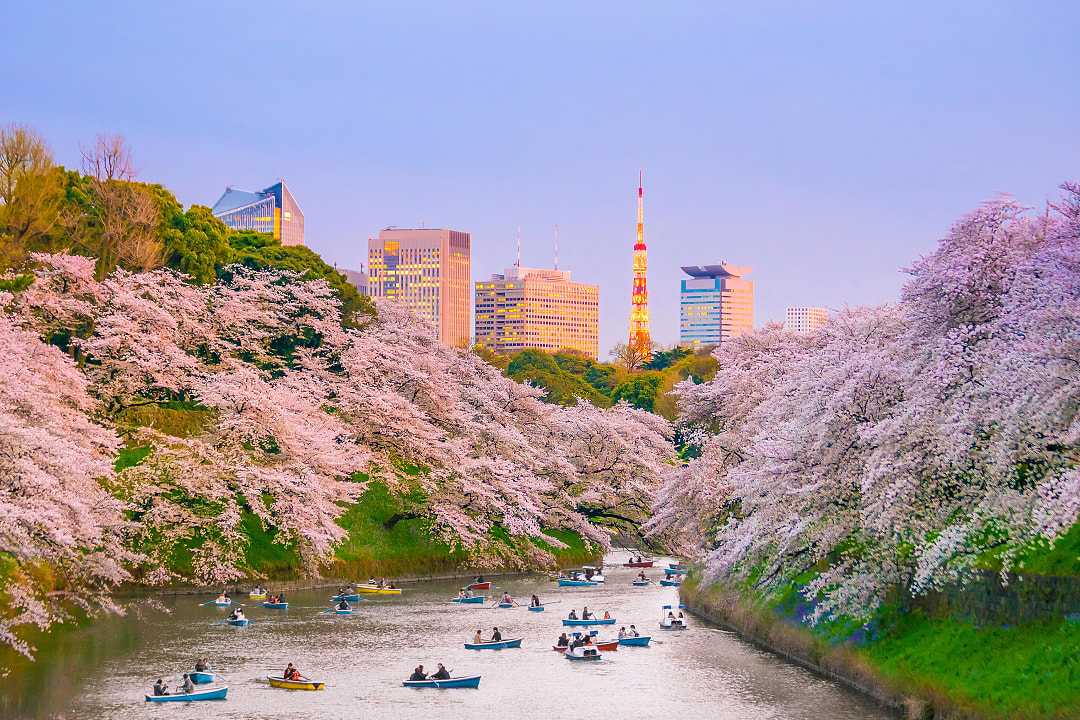This outdoor image showcases a river scene under a clear blue sky, with a touch of pink near the horizon where several multi-storied skyscrapers and a distinctive tower with orange, yellow, and pink hues stand. The river, appearing slightly murky and brown, flows away from the viewer, curving to the right, and is bordered by cement embankments. The green shores on both sides are adorned with vibrant, flowery vegetation, possibly lilacs or purple blossoming trees, cascading down the hillsides and nearly touching the water. The river is bustling with activity, as approximately 20 kayakers and boaters maneuver through the water, most in pairs and equipped with paddles. In the distance, more trees with brown and green foliage rise above the hills, blending with the colorful architectural skyline.